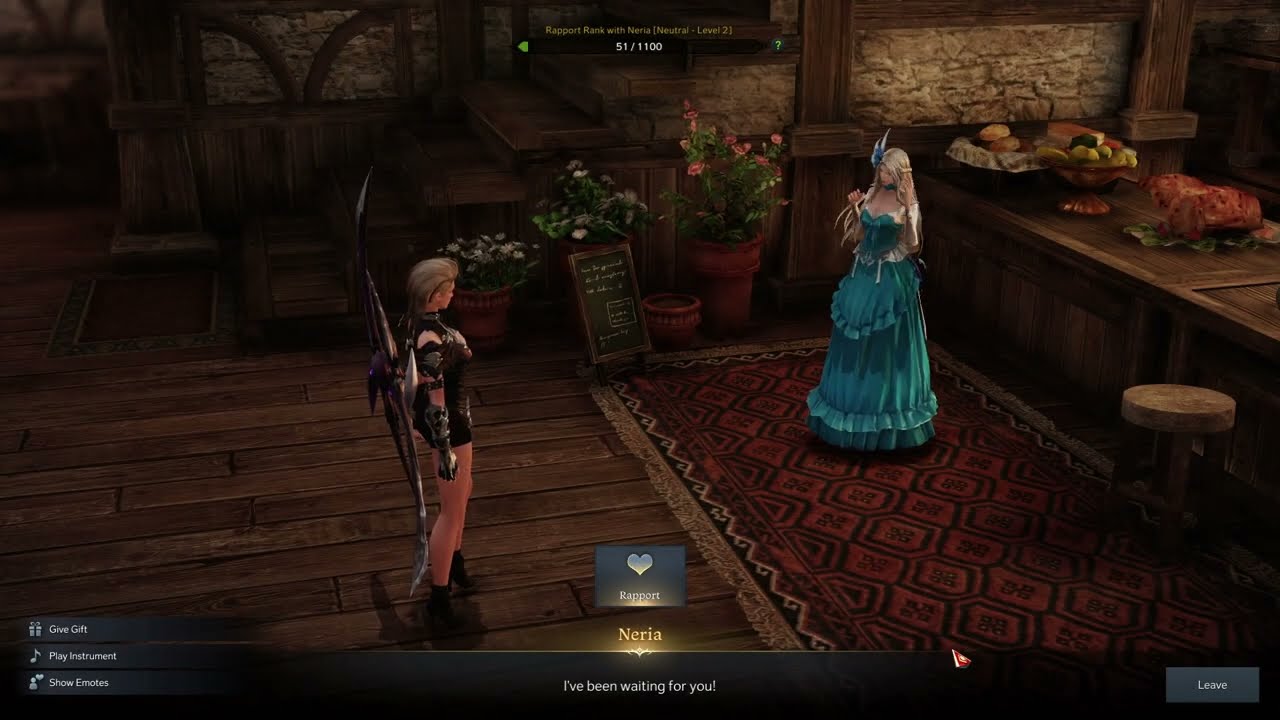This detailed screenshot captures a scene from a realistic, computer-generated video game set in what appears to be a medieval castle or grand hall, featuring rich wooden floors and intricate stone walls. In the image's dining area, the dark, rectangular wooden floor contrasts with a plush red and gold rug accented in dark purple or black, located on the right side. Standing on the wooden floor appears to be a character resembling a prince, featuring light-colored hair, wearing a dark brown leotard or tunic with attached armor, paired with dark shoes and a weapon, likely a bow of some sort, slung across his back. On the ornate rug, another character, seemingly a princess named Nerea, based on the illuminated text at the bottom center, wears a flowing turquoise gown and has long blonde hair. She stands near a wooden bar or banquette, which is laden with various foods such as fruit, bread, and meat. The princess has one hand raised to her head and the other holding an object possibly resembling a scepter or weapon. Additional details include multiple pots with flowers and a blackboard with white writing at the center of the room. The gameplay interface elements, such as a black strip with the text "I've been waiting for you!" and various control icons, suggest an immersive, story-driven game in a medieval-inspired setting.